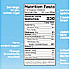In this image, set against a predominantly white background, there is a very small, grainy, and almost illegible label that appears to display nutritional facts. The label is ensconced within a light blue square, featuring a central white rectangular box with black lettering that reads "Nutrition Facts." Though difficult to decipher, it seems that the calories per serving are either 220 or 350, due to conflicting reports. Beside the central label, there is sparse white text on both the left and right sides against the light blue background. On the top left, there are approximately three lines of writing, followed by five lines below it. On the top right, there are four lines of text that appear to be cut off, with additional cut-off text below comprising three and then six lines of information. Despite much of the text being too small to read, it is clear the label is providing detailed dietary information common to food packaging.